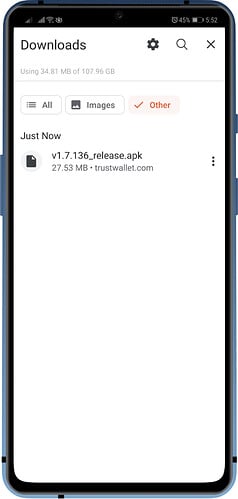The image displays a smartphone screen, presumably in a downloads section or settings menu. At the top of the screen, a black status bar includes several icons: a wireless signal icon, a Wi-Fi symbol, an indeterminate icon, a clock symbol, and a battery indicator showing 45% charged. The current time, 5:52, appears in the upper right corner.

Below the status bar, the main interface shows various elements. Near the top, a gear icon indicates settings, flanked by a magnifying glass for search functionality and an "X" button, likely for closing the current menu. Just beneath, a sentence reads, "Using 34.81 MB of 107.96 GB," indicating current storage usage. Below this, there are filter buttons labeled "All," "Images," and "Other," with "Other" currently selected.

Further down, under a "Just now" timestamp, an icon resembling a page appears next to the file name "v1.7.136_release.apk," which is 27.53 MB in size and downloaded from trustwallet.com. Adjacent to this file description are three vertical dots, likely representing additional options.

The entire display features a white background with black lettering, maintaining a simple yet functional aesthetic. The image overall captures what one would see if holding the phone and reviewing their recent downloads or exploring the settings menu.